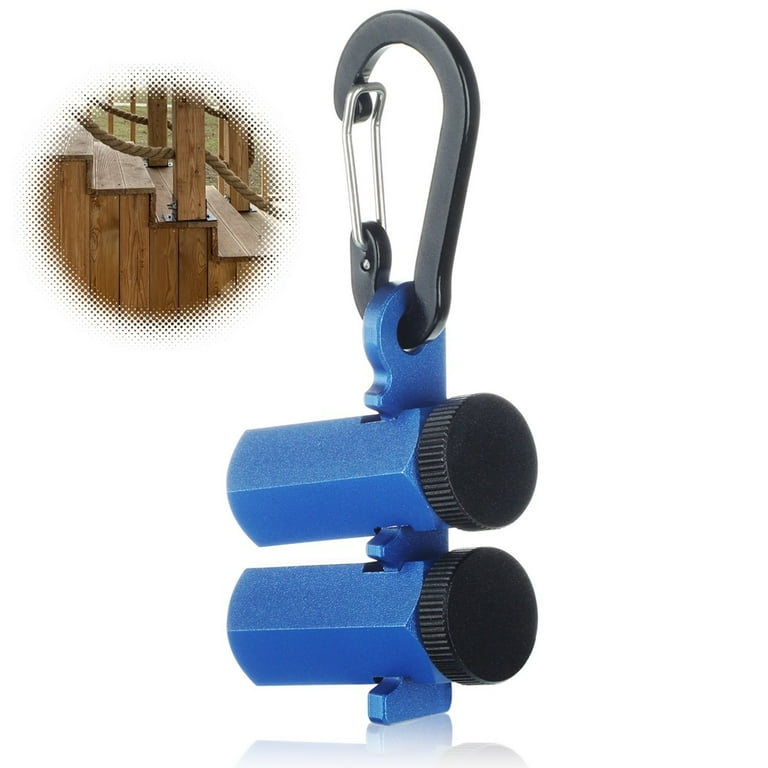The image depicts a complex device featuring elements of a carabiner with a large gray hook at its core. Attached to the metal hook is a blue plastic section connected to two black plastic caps with textured edges. Emerging from these caps are plastic tubes, collectively forming an intricate mechanism. To the upper left of the main device, there is a partially seen inset featuring a circular image of wooden steps with rope railings, surrounded by bubble-like circles. The device appears to lack any textual labels, making its purpose unclear. The detailed representation includes distinct geometric shapes and materials, combining metal, plastic, wood, and rope into a visually intriguing composition.